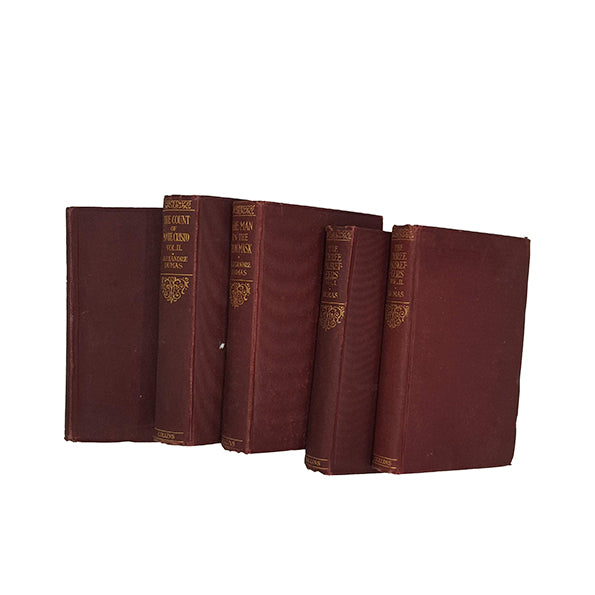The image features five classic maroon leather-bound books set against a plain white backdrop. These books are distinguished by their elegant gold lettering and decorative designs along the spine. Each book displays a slightly different shade of reddish-brown, contributing to an overall appearance of age and timelessness. Titles such as "The Count of Monte Cristo" and "The Man in the Iron Mask" can be discerned, hinting at their classic literary origins. The spines, adorned with intricate gold text and motifs, are mostly facing to the left, though the book on the far left is positioned differently, obscuring its spine text. The absence of book jackets highlights the vintage maroon leather and unified gold detailing, suggesting they might belong to a collection or series, possibly by the same author, potentially Alexandre Dumas. The minimalist setting, without any additional background elements, focuses all attention on the timeless beauty of these well-preserved literary works.